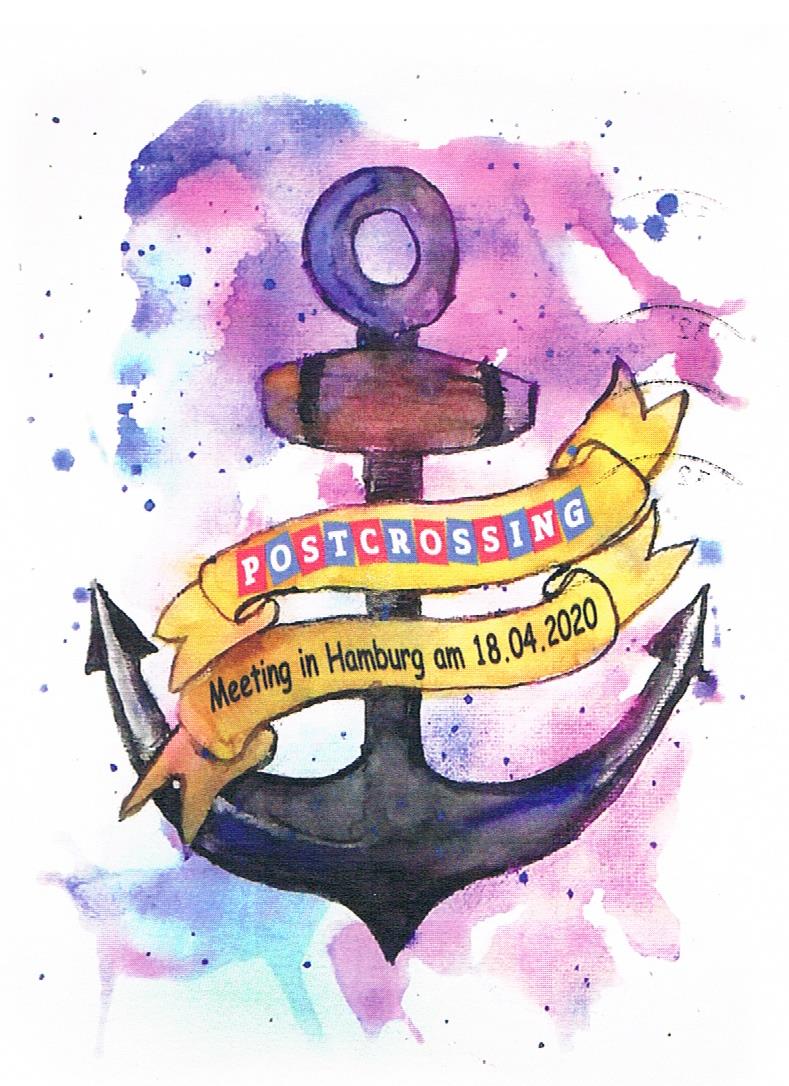The image features a vibrant watercolor-style artwork of a vintage ship anchor set against a white cardstock background with a tie-dyed pattern of pinks, purples, and blues, creating a vivid backdrop. The anchor itself is depicted in black with highlights suggesting reflections. Two yellow banners cross the anchor at diagonal angles. The top banner has the text "Post Crossing" written in alternating blocks of pink and blue with white lettering. The lower banner, written in black, reads "Meeting in Hamburg AM 18.04.2020." The overall composition is colorful and dynamic, evoking a sense of maritime tradition blended with contemporary art style.